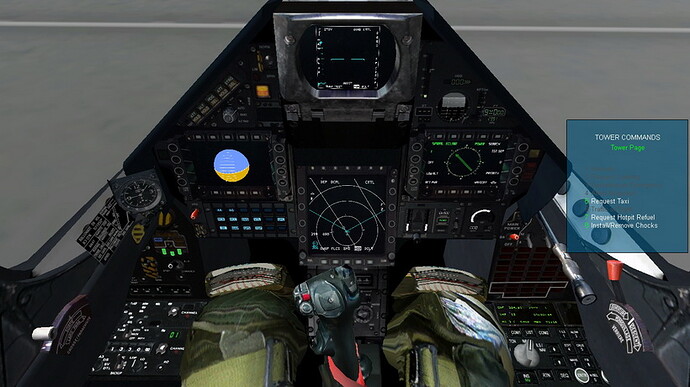The image depicts the control panel of a jet or fighter aircraft, resembling a video game interface rather than a real-life view. A semi-transparent blue overlay screen on the right reads "Tower Commands" in white capital letters at the top, followed by "Tower Page" with options below such as "Request Taxi," "Request Hot Pit," "Refill," "Install," and "Remove Chocks." The triangular-shaped control panel, filled with various graphics and buttons, is set against the tarmac of an airport with a white stripe visible in the background. In the foreground, a joystick sits between two green-gloved hands, with the pilot's green pants and knee pads visible on either side. The panel is mostly dark grey and black, featuring multiple screens, graphic displays of the horizon, and numerous buttons and knobs, all situated above a grey background.